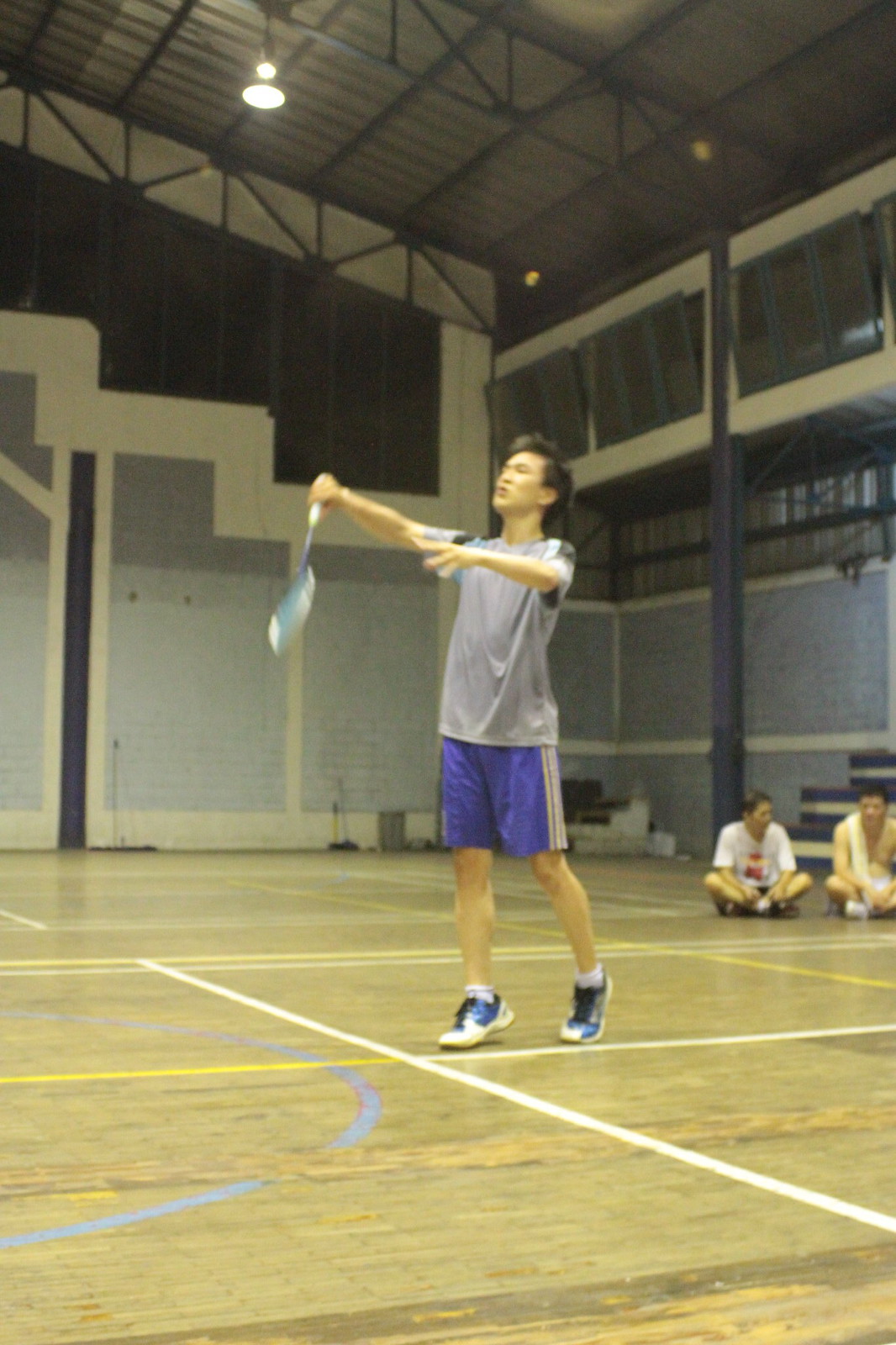The photograph depicts a young person of oriental features, likely a high school student, playing badminton inside a brightly lit gymnasium with a tall ceiling supported by iron bars. The subject, who has a light skin complexion and short black hair, is captured mid-action holding a badminton racket in his right hand. He is dressed in blue shorts with white stripes, a grey t-shirt, and blue sneakers with white accents. The gymnasium's wooden floor, marked for multiple sports including basketball and badminton, features white, yellow, and blue tapes designating the different courts. The walls are painted grey at the bottom with thick yellow stripes above. In the background, two individuals sit cross-legged on the floor, possibly waiting for their turn to play. The photo is vertical and clearly illuminated by the overhead indoor lighting, contributing to the overall bright and clear setting.